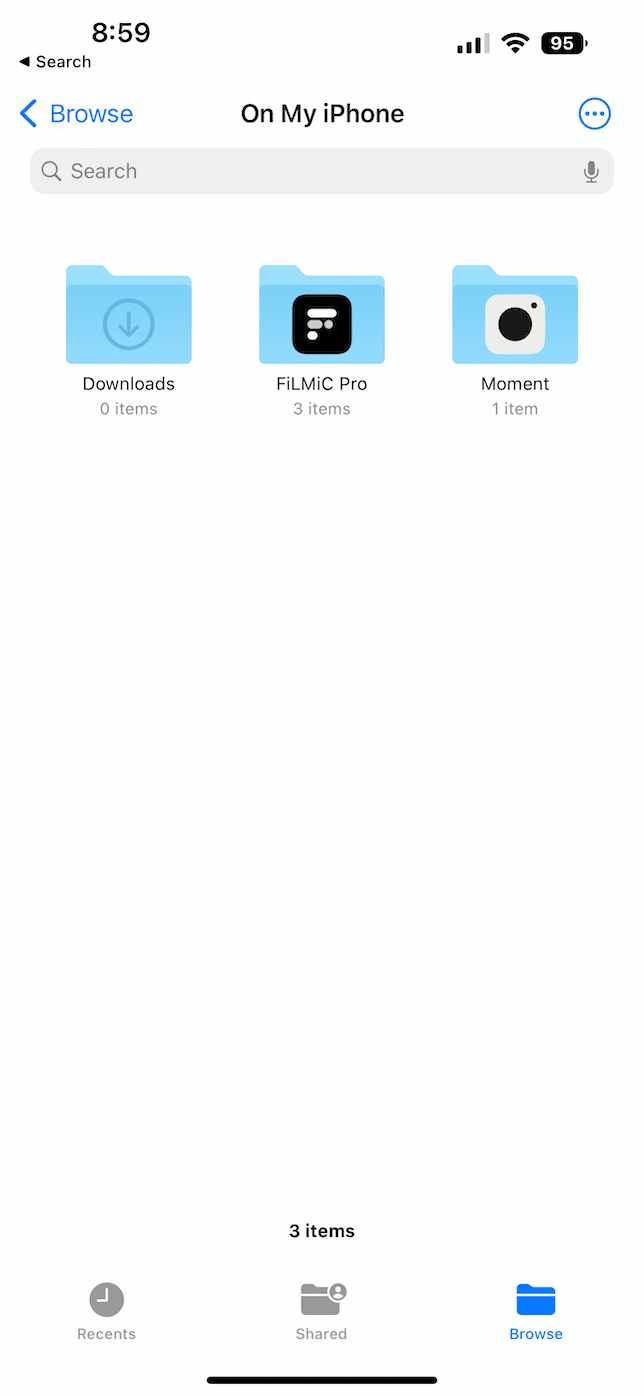The image displays an iPhone screen with various interface elements. At the top left corner, the time reads "8:59" followed by the status indicators on the top right: a wireless signal icon, a cellular connection icon, and a battery icon that is mostly full with "95%" inside it.

Below the status bar, there's a navigation bar with white text. On the left, it says "Search" with a left-pointing arrow, and on the right in blue text, it says "Browse," also accompanied by a left-pointing arrow. Centered on this bar is the text "On My iPhone." Adjacent to this on the far right is a blue circle containing three horizontal blue dots.

The next section features a search bar with a gray background. On the left side of this bar, there is a magnifying glass icon followed by the word "Search," and on the far right, there is a microphone icon.

The main section of the screen has a white background featuring three blue folder icons arranged side-by-side. The first folder shows a circle with a downward arrow inside it, labeled "Downloads" with "0 items" underneath. The second folder has a black square inside it and is labeled "Filmic Pro" with "3 items" underneath. The third folder, on the right, has a camera icon inside it and is labeled "Moment" with "1 item" beneath.

At the bottom of the screen, a footer bar presents three icons. On the far left, there is a clock icon with the label "Recents," in the center, a folder icon labeled "Shared," and on the far right, a blue folder icon labeled "Browse." At the very bottom, it reads "3 items."